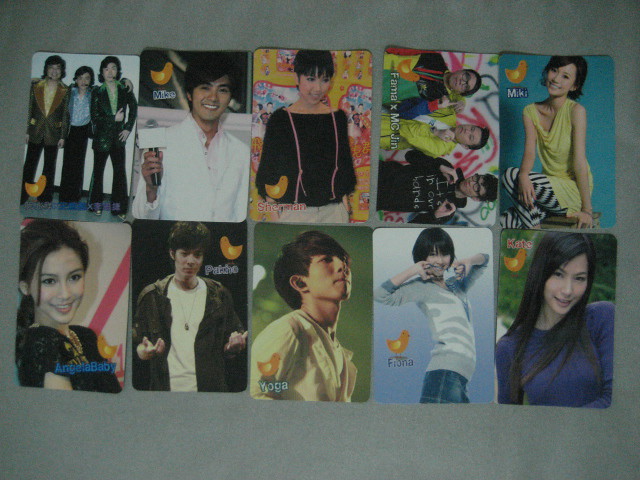The image showcases a diverse collection of cards, each featuring various individuals who appear to be of Asian descent. The topmost card on the left presents three men donning suits and jackets, typical of the 1970s style, exuding a sense of retro charm. The following card captures a young man beaming with a smile, dressed in a white jacket and holding a microphone, suggestive of a performer or host. The third card depicts a woman in a black blouse paired with white pants, her short bangs framing her face. Next, the fourth card displays three young men clad in vibrant, colorful outfits, possibly hinting at an artistic or musical background. Finally, the fifth card features a slender woman in a sleeveless orange blouse combined with white and black striped pants. The ensemble of cards collectively conveys an impression of notable personalities, potentially celebrated figures in the realms of art, sports, or media.